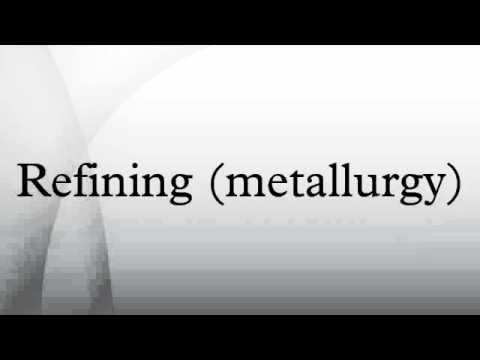The image depicts a minimalist title page, likely from a presentation or academic work. The design features a black border at the top and bottom of the page, with none on the sides. The main background transitions from dark gray at the bottom to almost white near the top, intersected by subtle horizontal bands and arcs of varying gray tones. The centerpiece of the page is black text, positioned in the middle. The text reads "Refining," followed by "Metallurgy" in parentheses. Overall, the page's simplicity and monochromatic color scheme give it an understated, formal appearance.